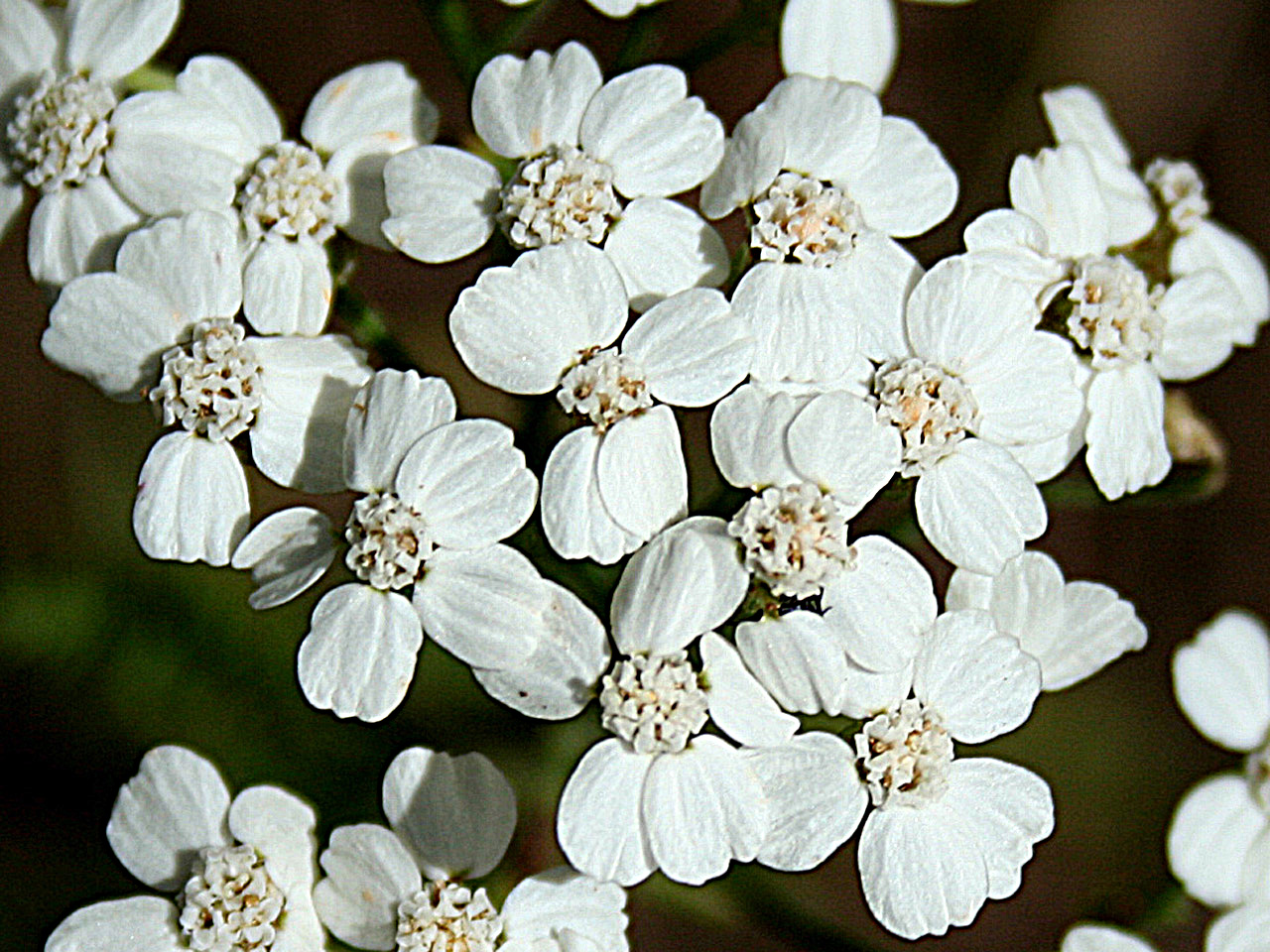This photograph features a close-up, top-view of approximately 15 white flowers, each with 4 to 5 round-shaped petals. The centers of the flowers are white and brown, containing visible reproductive parts with some pollen. The flowers are clustered mainly in the middle of the image, with some extending towards the top left, bottom, and right sides. The background is blurred, adding green and brown hues that hint at the natural surroundings. The rectangular image, taken in portrait orientation, has an almost square appearance and exhibits a low-quality, washed-out texture, making the flowers appear somewhat artificial.